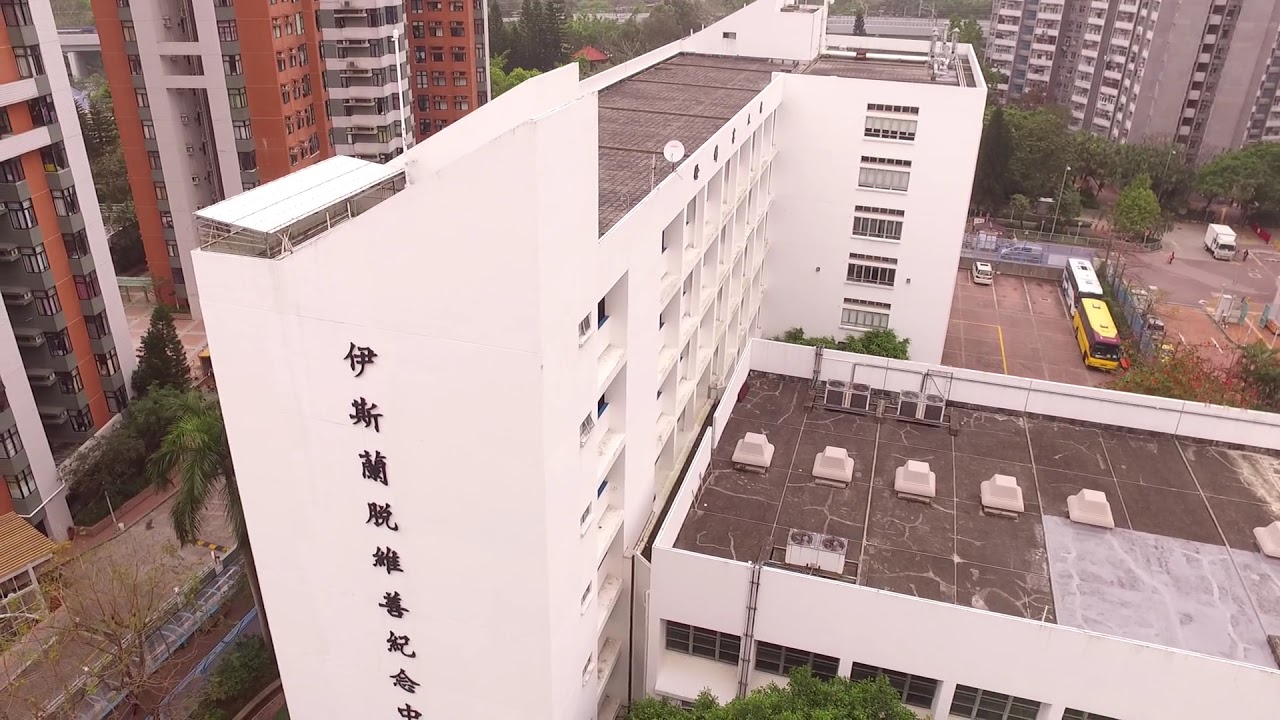The image is a horizontally aligned rectangular photograph taken from above, capturing an urban cityscape during the daytime. The central focus is a multi-story building—likely six or seven stories high—with an off-white facade adorned with a vertical series of black Asian characters, suggesting an East Asian location. Attached perpendicularly to this main building is a one-story structure characterized by a patchy brown rooftop with gray swirls, housing multiple air conditioning units. In the background, there's a parking lot occupied by two buses, one yellow and one white, along with other vehicles. Flanking the scene, particularly in the upper and lower left corners, are taller apartment buildings made of red brick and gray columns, some reaching up to 15 stories high. No people are visible, but several trees add greenery to the streets below.